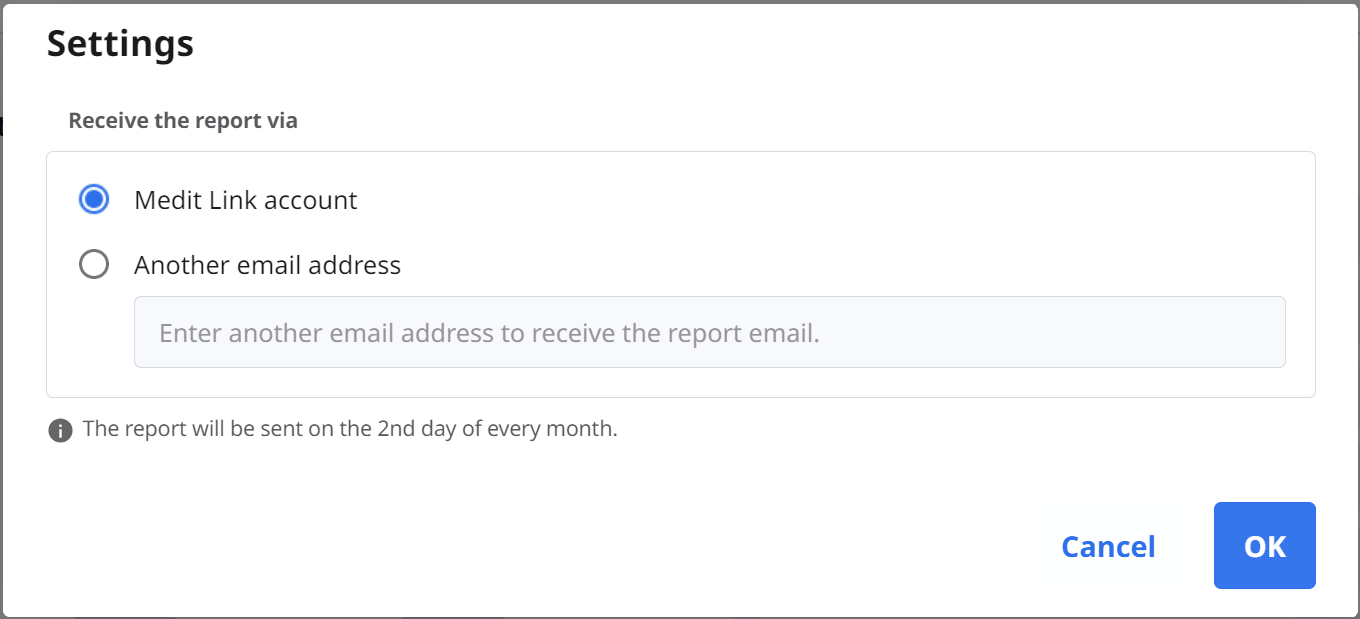The image portrays a settings window with a white interior and thin black borders. In the upper left corner, it is labeled "Settings." Below that, in black text, it reads "Receive the Report Via." Within this main box, there is a smaller white box with a gray outline that includes two radio buttons. The first radio button is selected and highlighted in blue, with the text "Edit Linked Account" next to it. The second radio button, unselected, is labeled "Under the Email Address." 

Beneath these radio buttons, there is a gray-outlined rectangular box, which contains darker gray text instructing the user to "Enter Another Email Address to Receive the Report Email." Below this text, positioned slightly outside the box, is a gray circular icon with a white lowercase "i" in the center, indicating additional information is available. Next to this icon, in dark gray text, the image notes, "The report will be sent on the 2nd day of every month," with "2nd" written using the numeral "2" followed by "nd."

At the bottom right corner of the window are two actionable buttons. The first button, in a faint white outline, is labeled "Cancel" in blue text with a capital "C." Adjacent to it, a blue button with white text displays "OK" in all capital letters.